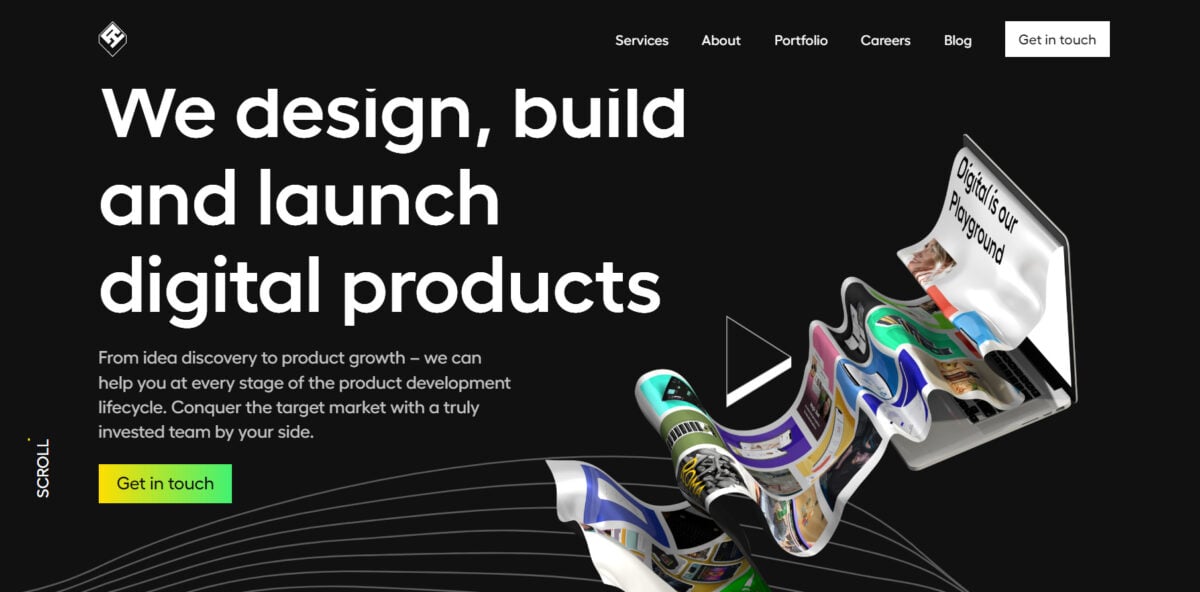The design website features a sleek black background, creating a modern and professional aesthetic. Prominently displayed in white font are the words "We design, build, and launch digital products." At the top right corner, the navigation bar includes links to "Services," "About," "Portfolio," "Careers," and "Blog." Adjacent to these links is a prominent white box labeled "Get in Touch."

Beneath the header, a comprehensive message reads: "From idea discovery to product growth, we can help you at every stage of the product development lifecycle. Conquer the target market with a truly invested team by your side." Below this text, there is a colorful, gradient box transitioning from yellow to lime green and then to green, also featuring the label "Get in Touch."

In the lower left-hand corner, the word "Scroll" is written vertically, guiding users to explore further. The website also includes a dynamic 3D design of their company emblem, depicted within a white box that contains black visual elements. Complementing this design is an intriguing visual of a printer. As paper flows out of the machine, the words "Digital is our playground" are printed on one sheet, while many others—displaying vibrant designs in purple, green, pink, and blue—cascade in various directions, creating a sense of motion and creativity.